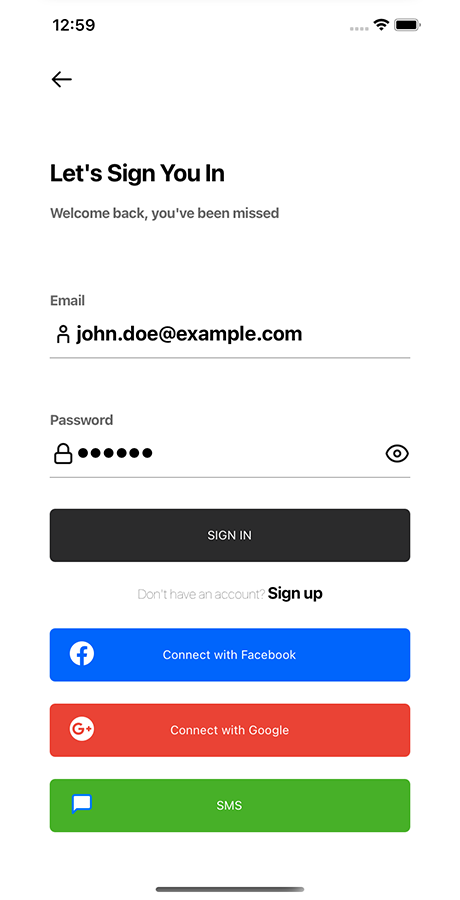Screenshot Description of a Sign-in Screen:

The screenshot captures a well-designed sign-in screen with a white background. At the very top of the screen, the status bar displays the time "12:59" in black text, accompanied by Wi-Fi and battery icons.

Below the status bar, there is a back arrow icon in black, indicating the option to return to the previous screen. Centered prominently is a welcoming message in black text: "Welcome back, you've been missed."

Beneath the greeting, there is a section to enter the user's email. An email input field is highlighted, with a placeholder text "Email" displayed beside a small person icon. The example email entered is "john.doe@example.com".

Directly below the email section, a thin gray line separates it from the password field. The password input area includes a small padlock icon and is masked with black circles for security. Adjacent to this is an eye icon, likely for the option to show or hide the password.

Following the password field, there is a prominent black box with white text reading "Sign In." Underneath this button, in smaller gray and black text, is the option for new users: "Don't have an account? Sign up."

Further down, the screen offers alternative sign-in options with three distinct boxes:
1. A blue box with the white text "Connect with Facebook," featuring a Facebook logo (a white circle with a blue 'F').
2. A red box with the white text "Connect with Google," accompanied by the Google+ logo (a white circle with a red 'G' and a plus sign).
3. A green box with the white text "SMS," including a logo of a white box with blue trim.

Finally, a thin gray line appears at the bottom of the screen, marking the end of the visible content.

This detailed layout ensures users can easily access and use the various sign-in options available.